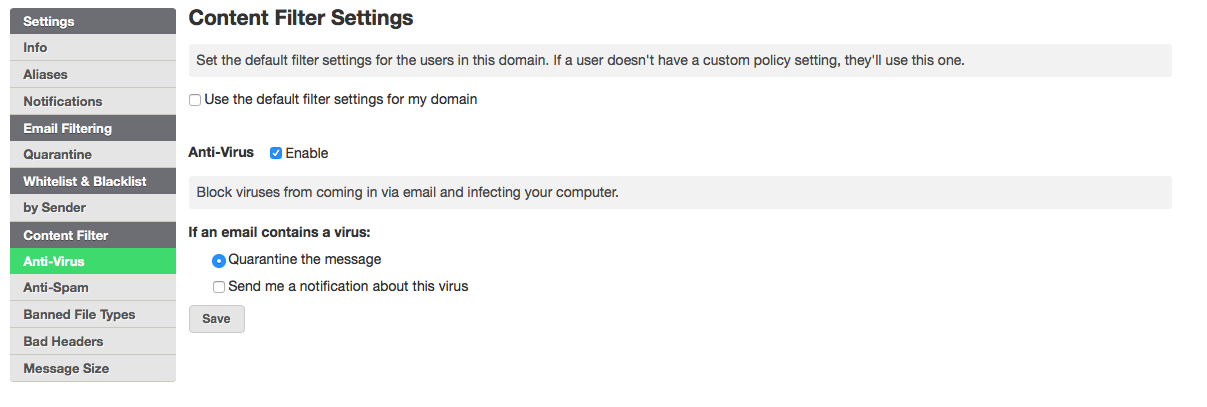Caption: 

A detailed grid interface shows various filter settings for managing user email preferences. The columns include options for "Settings," "Info," "Alias," "Notifications," "Email Filter," "Quarantine," "Waitlist and Blacklist by sender," "Content Filter," "Antivirus," "Antispam," "Bantala," "TimeSpam," "MrSign," and "Content Filter Settings." Users can configure the default filter settings for their inventory here. 

If no custom filter is set by a user, the system will default to these settings. An unchecked blue box under "Antivirus" indicates that email virus blocking is not enabled by default. Users can choose to quarantine any email containing a virus by selecting the option next to "Quarantine the message," while the notification setting remains unchecked, meaning no notification will be sent about the virus. 

The "Save" button is visible below these options. The background of the interface is white, with the "Antivirus" section highlighted in green to signify its status.